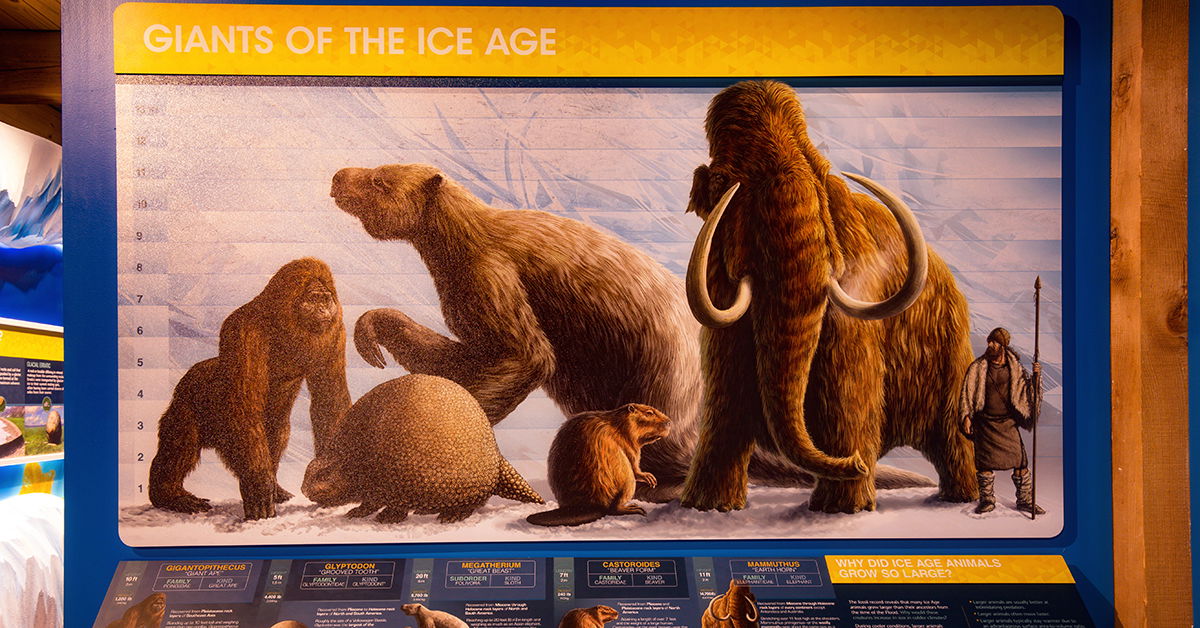The image depicts an informational display board similar to those found at the Museum of Natural History, titled "Giants of the Ice Age." This title is presented in white text over a prominent yellow horizontal banner at the top of the blue board. Below the title, there is a detailed drawing showcasing various extinct mammals from the Ice Age era. On the left side of the drawing stands a gazelle with notably long front limbs. At the center of the illustration is a large, furry animal, resembling either a gorilla or a bear, also with exceptionally lengthy front arms and facing leftward. In the forefront, a diminutive brown creature that resembles a mouse is depicted with short front legs. Beside it, slightly to the right, is an elephant-like animal with a coat of brown fur and tusks that curve upwards. Far right of the image stands a human figure dressed in brown attire, including a hat, a dress, and tall boots, holding a long stick or spear. All featured animals are illustrated in shades of brown, emphasizing their distinct sizes and features. Overall, the display captures the diverse and colossal fauna of the Ice Age, with a human figure for size reference to highlight the enormity of these ancient creatures.